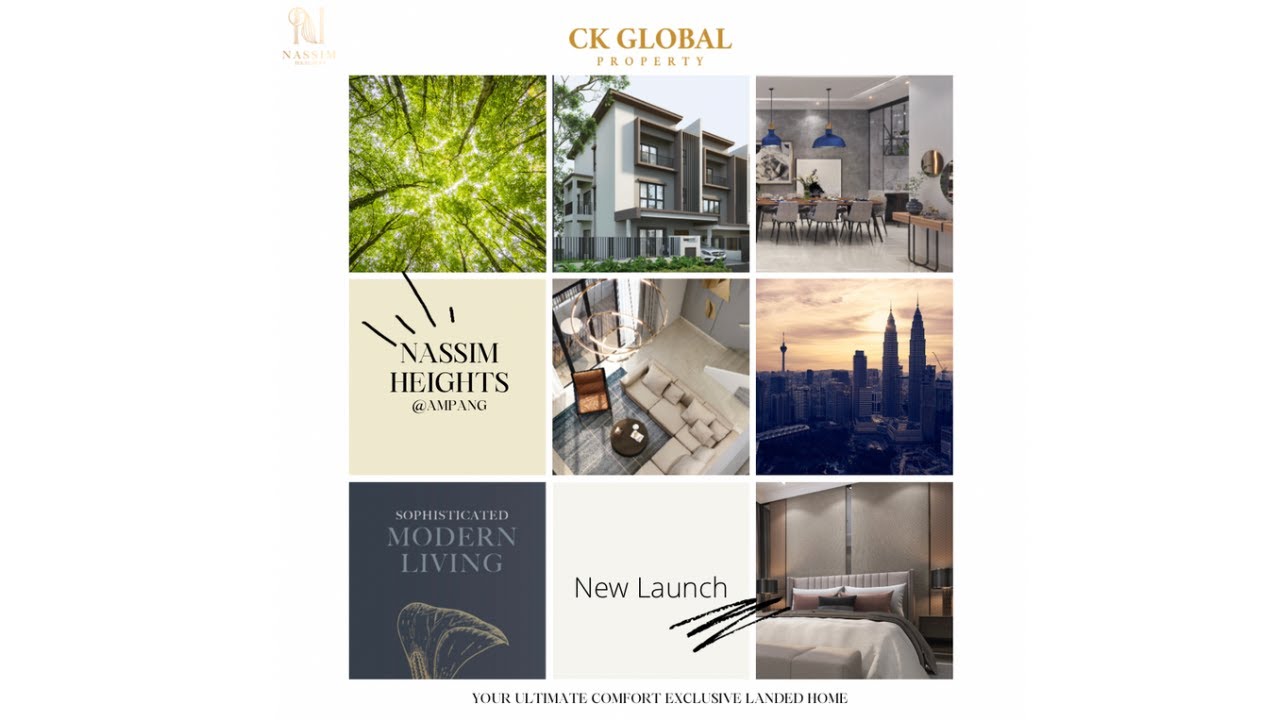**Caption:**
The image features a clean white background with "CK Global Property" prominently displayed at the top and "Your Ultimate Comfort: Exclusive Land and Home" elegantly written at the bottom. Arranged in a 3x3 grid, nine thumbnails showcase various aspects of the properties.

In the top-left thumbnail, a serene forest scene is captured, with the photographer looking upwards into the trees, creating a tranquil and natural ambiance. The adjacent thumbnail to the right depicts a modern apartment building, representative of urban residential options. The third thumbnail in this row provides an interior view of a stylish room, highlighted by blue light fixtures and a contemporary dining setup with a table and chairs.

The second row begins with an image on the left, marked by the text "Nassim Heights at Anpang," suggesting a high-end residential project in an exclusive location. The middle thumbnail offers a bird’s-eye view of a cozy living room, showcasing a comfortable couch and a sleek coffee table. The rightmost image in this row reveals a metropolitan skyline, presumably of Toronto, characterized by its distinctive buildings and a bustling urban feel.

The final row starts with a thumbnail on the left bearing the text "Sophisticated Modern Living," hinting at upscale and refined residential choices under the CK Global Property banner.